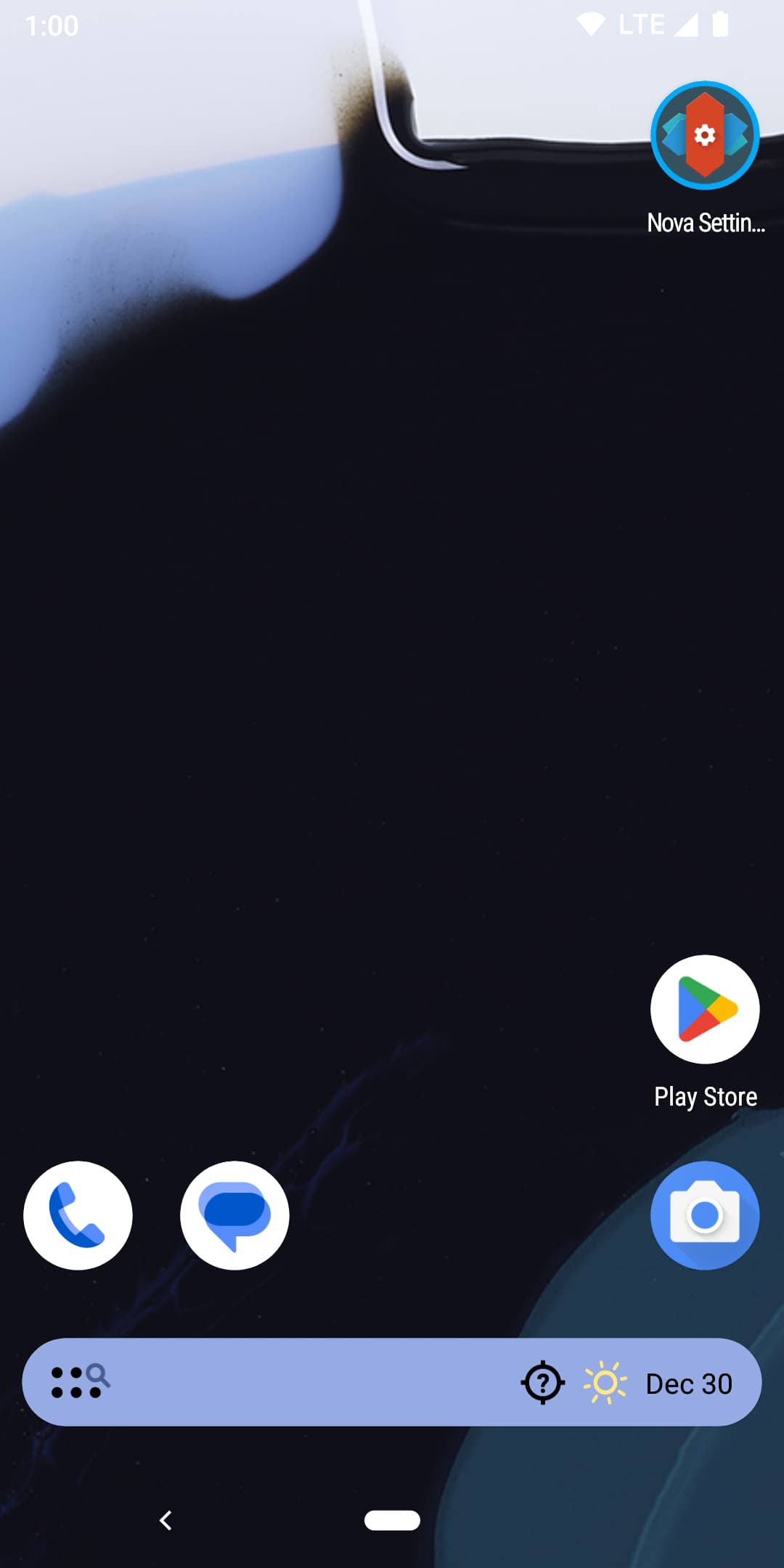**Detailed Caption:**

This is a screenshot of a mobile phone's home screen. The navigation bar at the top is a very light gray, making the white text and icons somewhat difficult to distinguish. It shows the time as 1 o'clock, with a full Wi-Fi signal indicator to the left. Next to the Wi-Fi icon, "LTE" is displayed alongside a fully charged battery icon.

The background image appears to be a poorly taken grayscale photograph of a mountain, with the majority of the image dominated by a large black blob that diagonally spans from the top right to the bottom left, covering about 80% of the screen. In the bottom right corner of the background image, a slate gray half-moon shape is visible.

Beneath the navigation bar on the upper right, there's an icon for Nova Browser labeled "Nova Settings," indicating it is for the Nova UI. Further down, occupying the bottom two-thirds of the screen, the Google Play Store icon and label "Play Store" are displayed. Aligning the bottom portion, from left to right, are the icons for the phone, SMS, and camera apps. 

At the very bottom of the screen, there's a blue search bar with the current weather information and date, specifically showing a sunny December 30th.